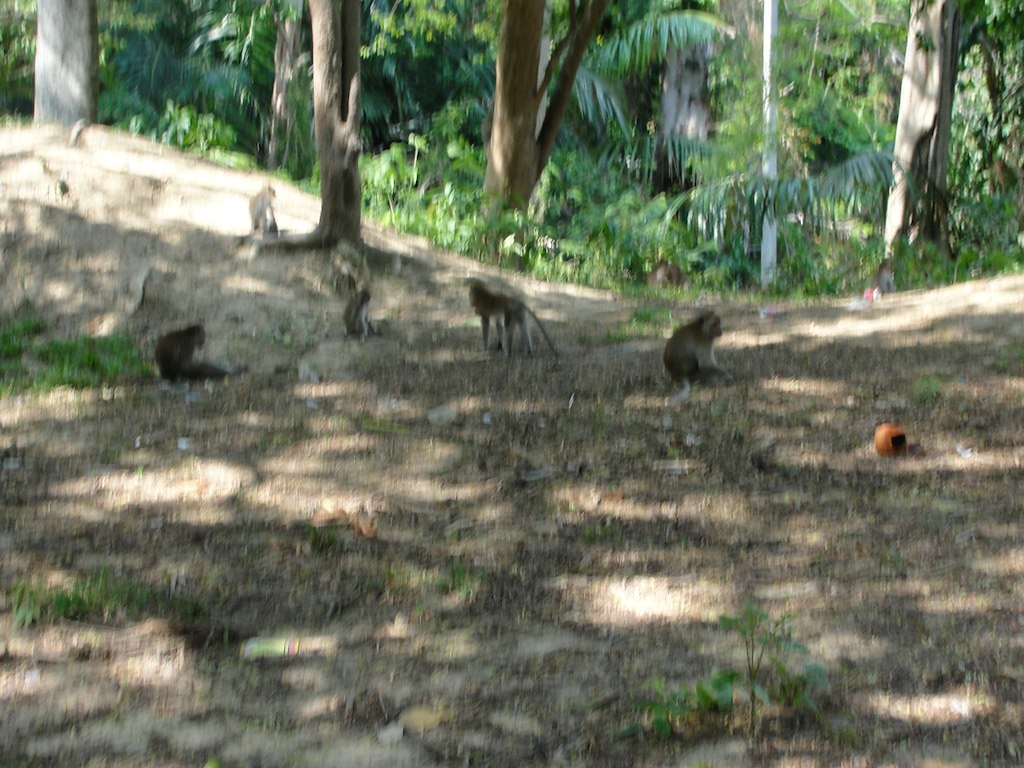This color photograph captures a shaded, tropical landscape filled with both flora and fauna. In the foreground, the ground is mostly brown dirt with patches of grass and plants. Scattered sunlight filters through the gaps in the foliage, creating spots of light on the ground. To the bottom right, a light brown monkey is sitting, gazing to the right. Additional monkeys are spread throughout the scene, although they appear blurry and out of focus. There are three clearly positioned next to the seated monkey, with one walking away and two sitting and looking to the right. A sixth monkey is partially visible in the background near a tree on the top left. Several tree trunks, predominantly brown, stretch upwards, and the area is enriched with lush green foliage, including palm fronds and other tropical plants. Among these natural elements, a mysterious cut-out pumpkin is positioned near the animals. The overall scene exudes a serene, natural environment, teeming with life and characterized by the dappled interplay of light and shadow.